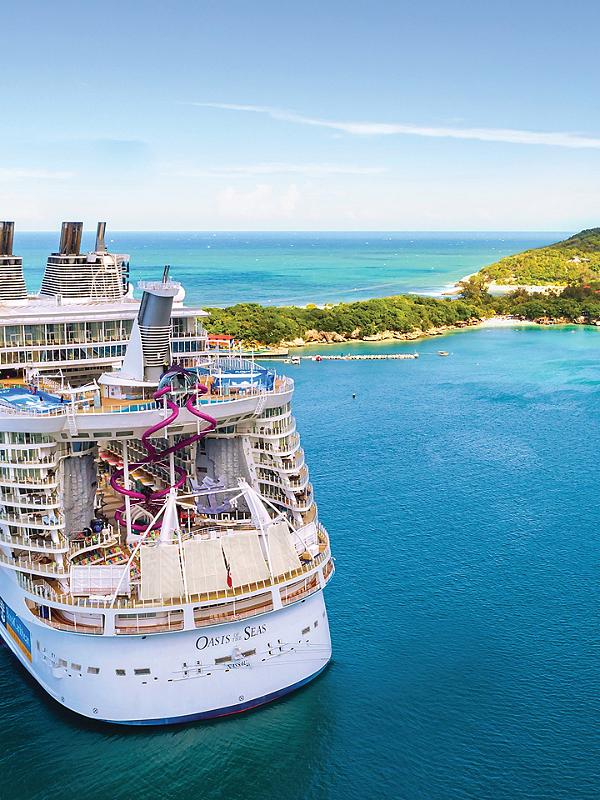This is a detailed photograph of the luxury cruise liner, Royal Caribbean's Oasis of the Seas, taken from a rear, elevated angle in vertical portrait orientation. The ship, predominantly white and immense in size with approximately eight to ten decks, occupies the left half of the image, appearing crowded with passengers. At the ship's center front at the top, a large smokestack is visible along with four chimneys and two prominent purple water slides that descend from the upper deck. Near these slides are swimming pools. The clear, crystal blue water around the ship looks inviting, contrasting with the small tropical island or sandbar to the right, which is narrow and extends about two-thirds across the photo. This piece of land is surrounded by more ocean on either side. Above the scene, a clear blue sky stretches across the horizon, adorned by a single black cloud, enhancing the tropical setting. The ship is positioned slightly angled to the right front, giving a comprehensive view of its luxurious exterior and features.